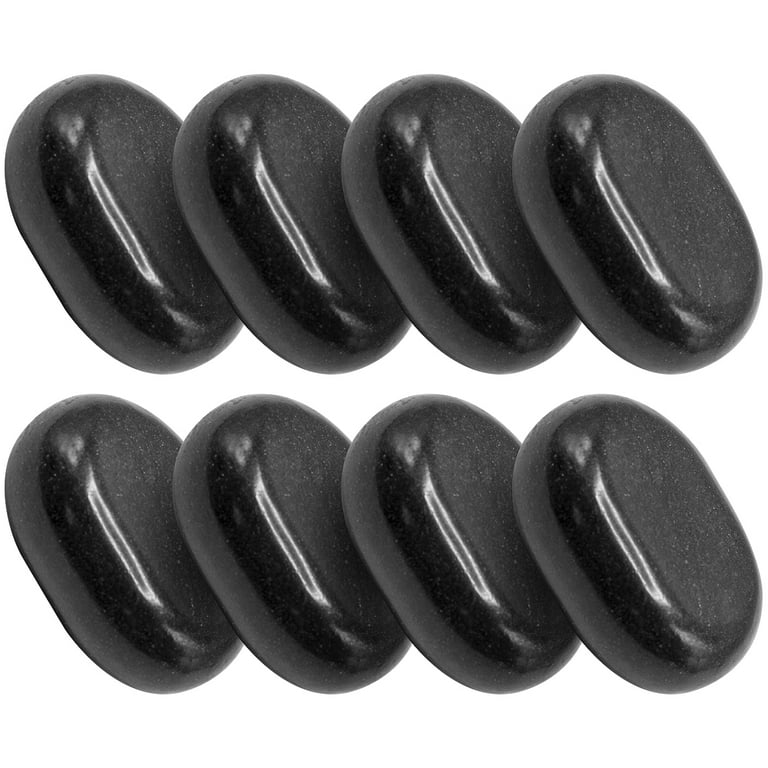The stock photograph features eight smooth, hand-polished black rocks contrasted against a solid white background. The stones are evenly divided into two rows of four, each perfectly aligned and placed next to one another with a small white gap separating the two rows. The rocks are cylindrical with flat, matte front and back sides, and highly polished, shiny edges that reflect light from the camera. Each rock is positioned at an angle, facing towards the right side of the image, giving a sense of uniformity and symmetry. Despite their simple and sleek appearance, the stones look identical in size and shape, potentially suitable for adornment, collection, or other decorative uses. The photograph effectively highlights the stones' glossy finish and precise arrangement, accentuating their aesthetic appeal.